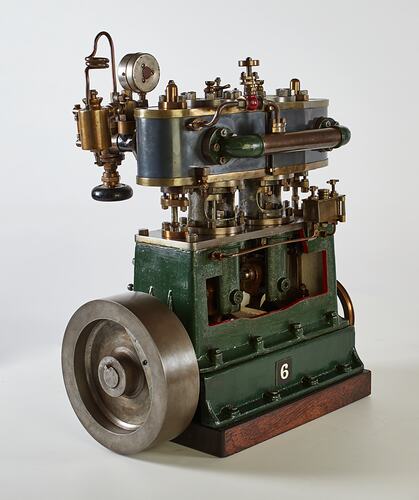In a stark, white room, the image depicts a complex and enigmatic piece of machinery. The base of this contraption is made of solid, dark wood, providing support for the structure above it. Rising from the base, the main body is painted a hunter green, reminiscent of a building's facade. Prominently displayed at the front is the number "6". On one side of the machine, a large, thick metal wheel is attached, which appears to be adjustable or turnable. 

The machine also features a variety of brass nozzles arrayed across its upper section, adding a golden hue to its predominantly green and brown color scheme. Positioned atop this green section is a royal blue upper part that seems to be the focal point of activity. This area is crammed with numerous tubes, knobs, levers, switches, and handles, all contributing to its intricate design.

The machinery includes shades of silver, green, blue, and gold, with occasional hints of red. Despite its detailed construction and color variety, the exact purpose of the device remains unclear. No explanatory text accompanies the number "6," leaving the function of this contraption to the imagination. The overall composition is slightly slanted, with the device centrally framed in the photograph.